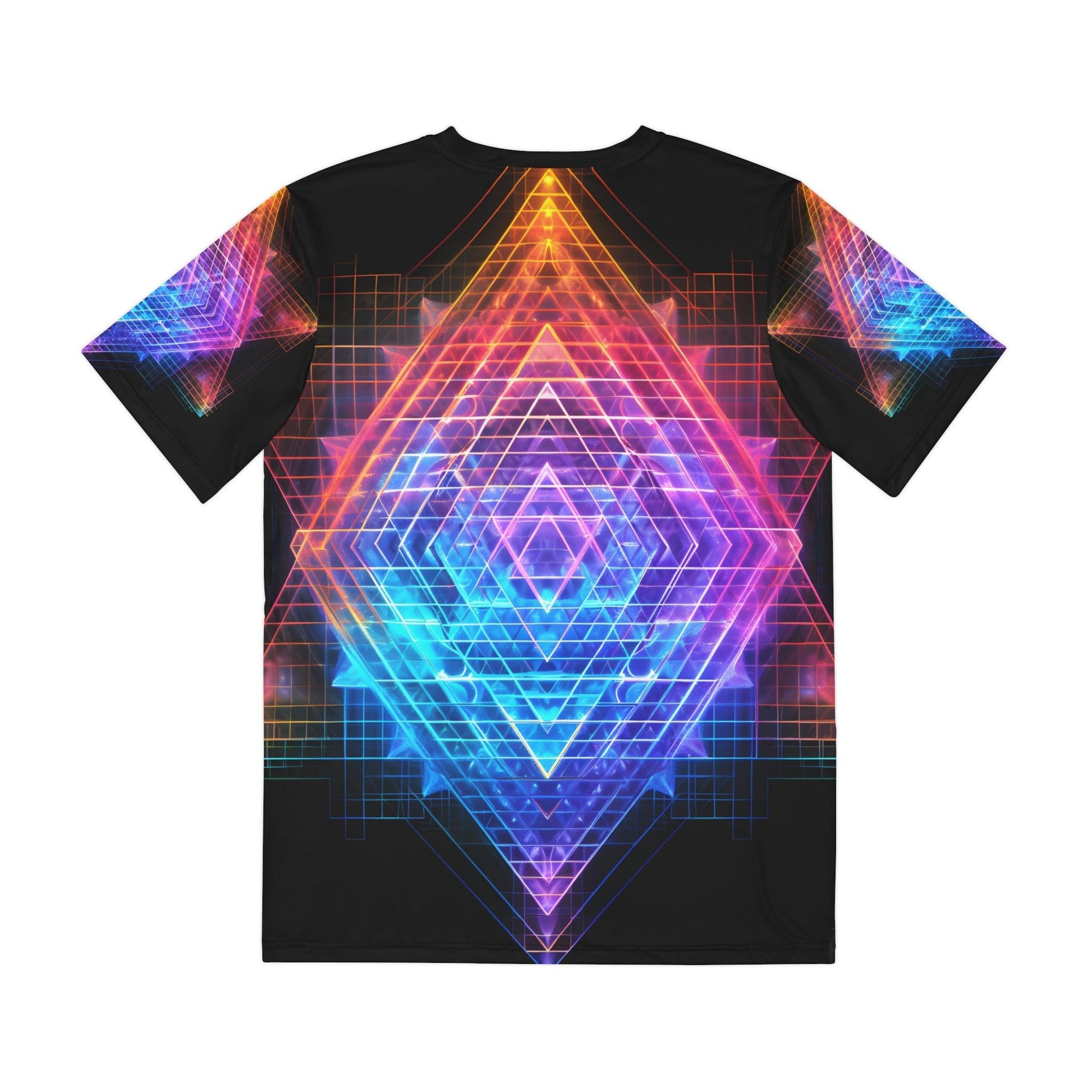This image displays a striking black short-sleeved t-shirt set against a pure white background. The centerpiece of the t-shirt features a large geometric design that begins at the neck and extends all the way down to the bottom of the shirt. This design is characterized by a diamond shape composed of progressively smaller and interlocking triangles. The vibrant colors in the diamond range from orange, red, and gold at the top, transitioning through pinks, purples, and blues to a deep electric blue at the bottom.

Behind the diamond, there is a grid-like pattern of small squares in matching neon hues, creating a textured backdrop that complements the central design. The same intricate geometric pattern, albeit on a smaller scale, is also present on each sleeve, extending from the shoulder to the end of the shirt sleeve. This visually stimulating design evokes a sense of video game aesthetics due to its vivid colors and complex graphic elements.